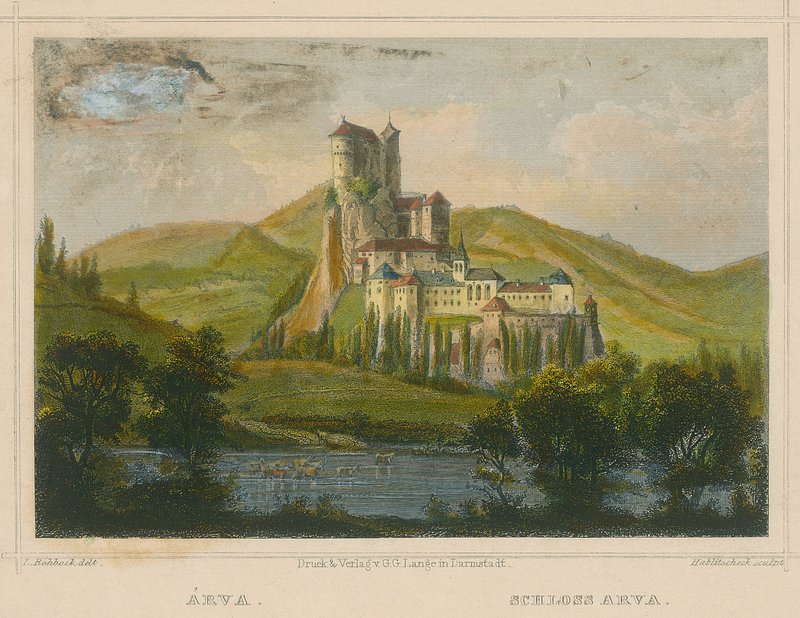The image depicts a vintage painting that resembles an ancient postcard from a bygone era, potentially the 1400s. The central focus is a medieval, white castle adorned with multiple red and blue rooftops and numerous turrets. The castle is situated partly on a hill and partly at a lower level near a serene blue river. This body of water, described variably as a lake or river, runs in front of the castle, surrounded by lush greenery and a variety of trees, some of which cast shadows suggesting minimal sunlight.

The landscape is set in a picturesque, mountainous region with green rolling hills in the foreground and background, enhancing the overall natural beauty around the castle. The sky above the scene is predominantly blue with scattered white fluffy clouds, yet there are some dark cloud formations in the top left corner, adding a touch of mystery.

The painting surface appears to resemble parchment, outlined by ancient-looking text written in an unidentifiable, old-fashioned script that hints at the artwork’s historical significance. The combination of the castle's layered structure with its various levels rising up the hill, the surrounding verdant landscape, and the tranquil water body makes for an enchanting and timeless scene that captures the essence of medieval tranquility and grandeur.